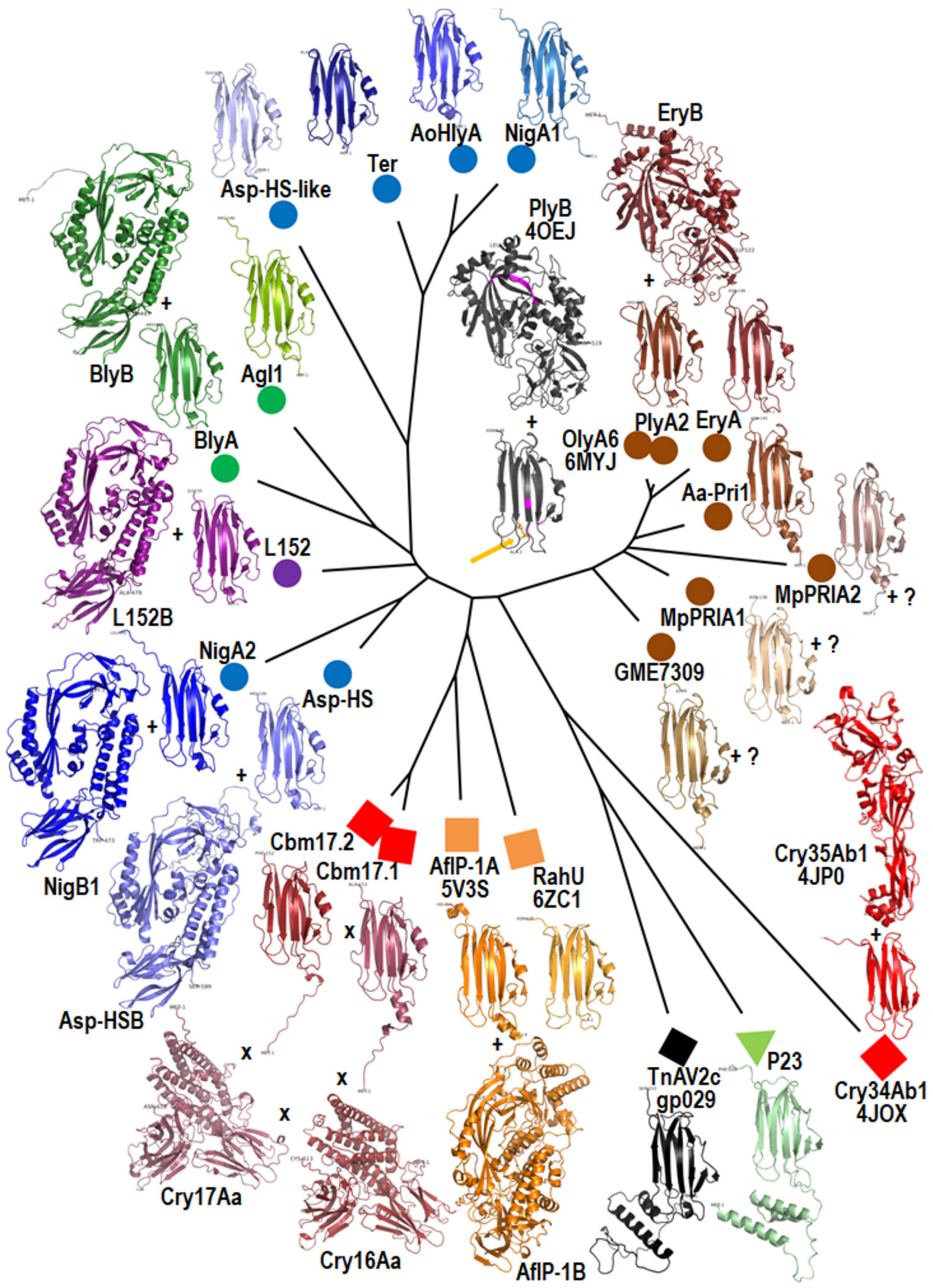The image is a detailed computer-generated diagram showcasing various protein structures. Central to the image is an arc from which several black lines radiate outward. At the end of each line is a distinctive ribbon-like pattern, each rendered in different colors such as blue, green, purple, light purple, red, orange, black, brown, bronze, gold, champagne, and copper. Accompanying each of these intricate patterns is a chemical name, signifying different proteins and their structures, such as ASP-HS-LIKE, TER, AOHIYA, NIGA1, ERYB, PLYB, AGL1, L152, NIGA2, CRY34AB1, and many more. Each protein structure is denoted by multicolored coiled shapes, indicating distinct protein compounds formed by specific combinations of amino acids. Additionally, a color-coordinated circle, often matching the respective pattern's color, is placed nearby each structure. Towards the bottom of the image, a series of shapes, including red squares, a black square, and a green triangle, further elaborate the protein formations and connections.